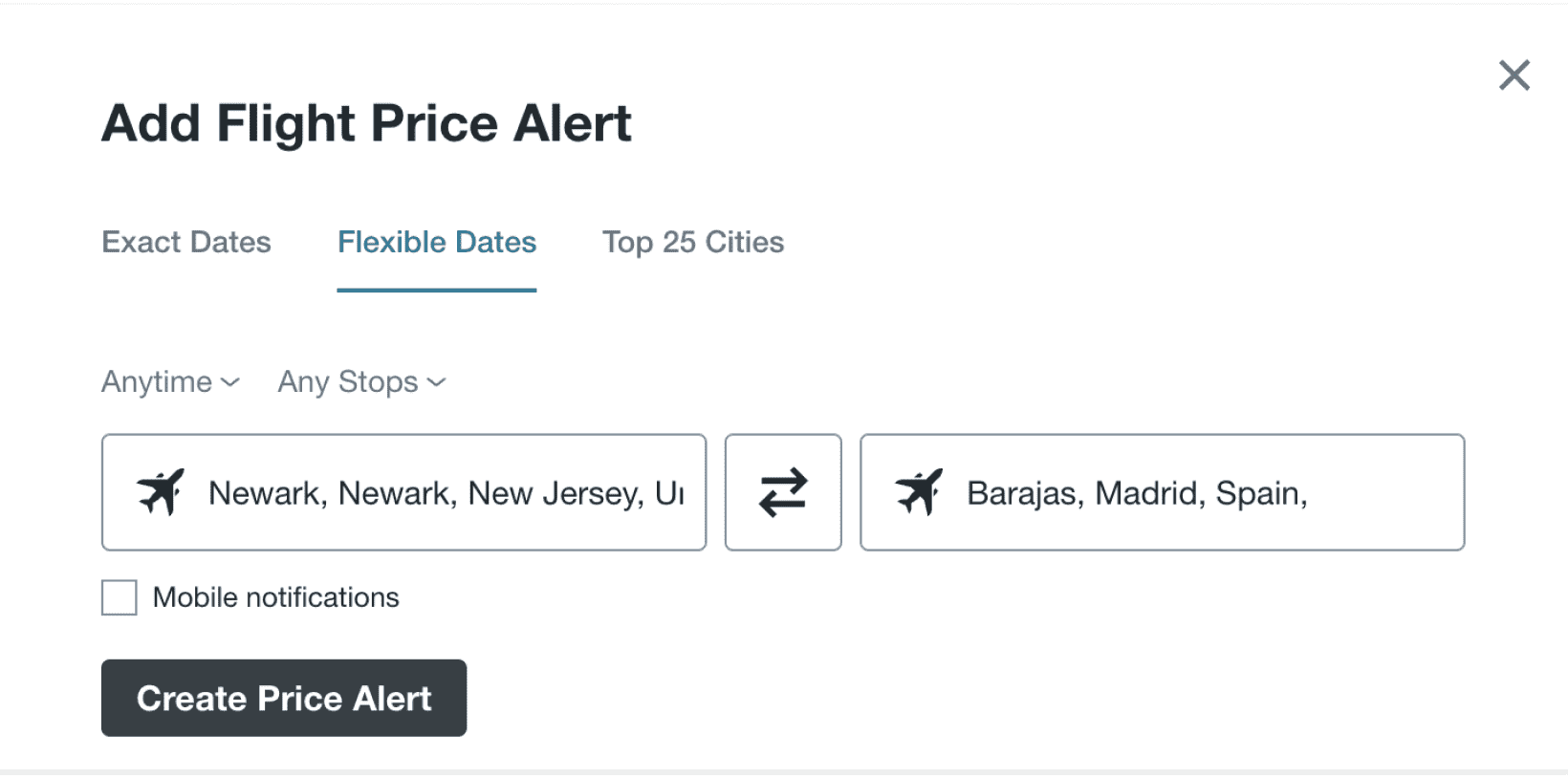The image features a user interface with a white background. In the top-left corner, there is a black text label that reads "Add Flat Price Alert." In the top-right corner, there's an "X" icon for closing the interface. Under the "Add Flat Price Alert" label, it reads "Exact Dates," and to the right is the "Top 25 Cities" option. Positioned in the center is "Flexible Dates," which is highlighted in a bluish-gray color with a horizontal line underneath.

Below these options, there is a section labeled "Any Time" accompanied by a drop-down menu. Adjacent to this on the right is another drop-down menu labeled "Any Stops." Beneath these menus, there's a rectangular text box with an airplane icon and the label "Newark, Newark, New Jersey." Next to this, on the right, is a square with left and right arrows. Further to the right is another rectangular text box with a plane icon labeled "Barajas, Madrid, Spain." At the bottom of this interface, there's a square labeled "Mobile Notifications."